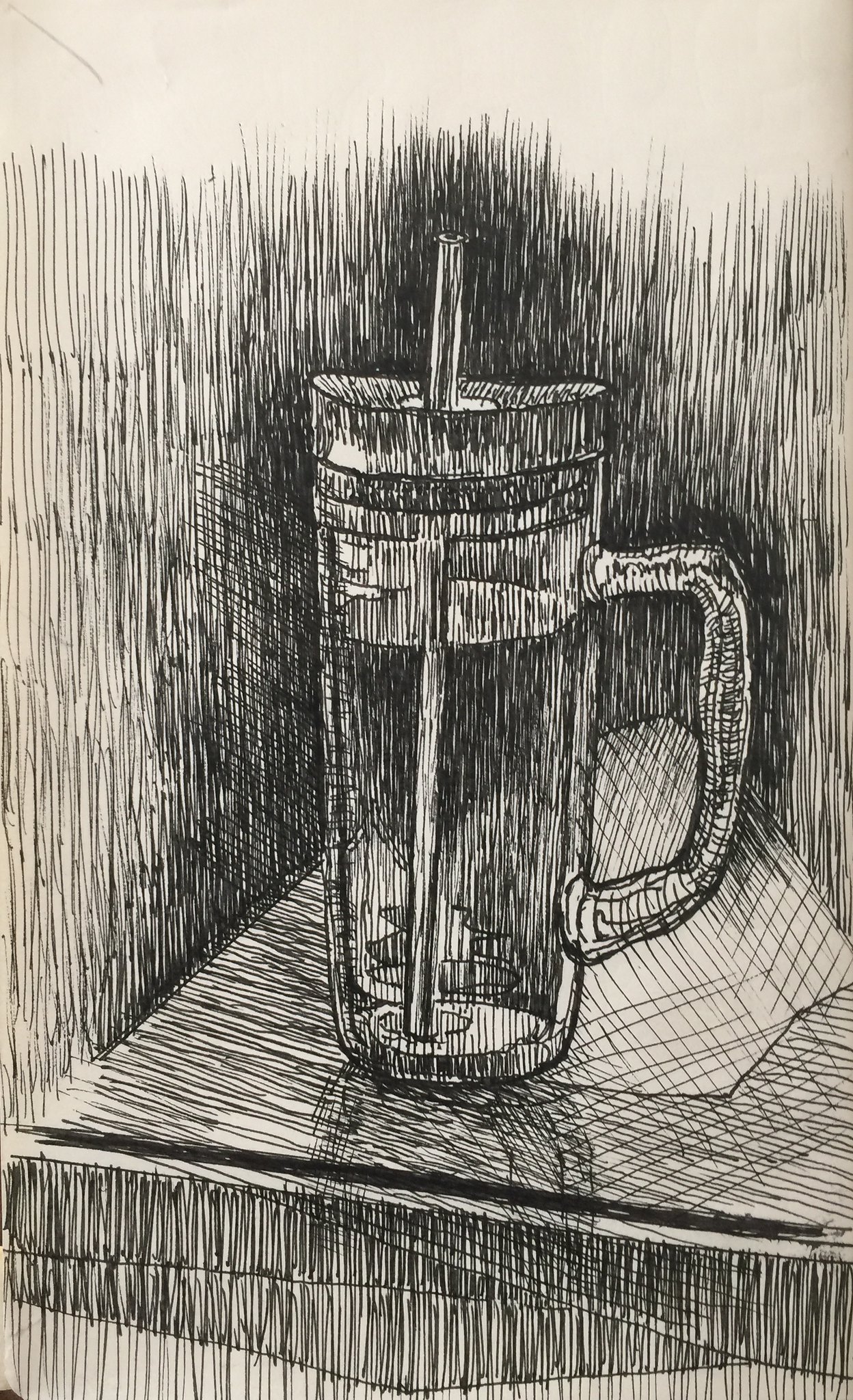The image is a detailed pencil drawing of an oversized cup with a prominent handle, featuring a straw that pierces through its middle. The cup, which resembles a large glass of water, is positioned on a table. The entire composition is executed with delicate, thin lines typical of pencil artwork, and the monochromatic palette accentuates the fine details of the illustration. The cup casts a dark shadow on the table surface, adding depth and realism to the scene. Additionally, there appears to be a lid atop the cup, enhancing its resemblance to a large mug. The artwork is rendered on white paper, highlighting the contrast created by the meticulous pencil strokes.